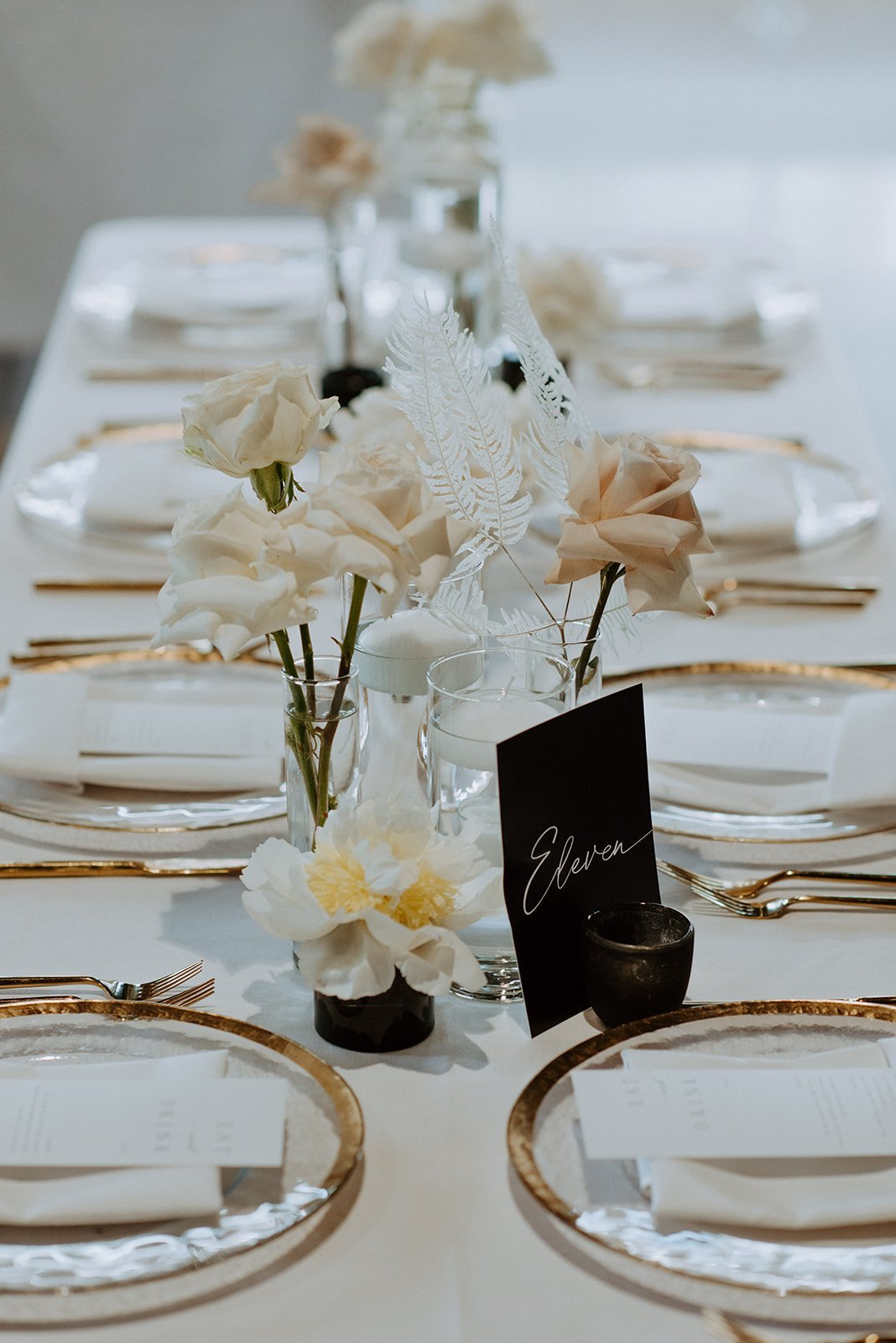The image depicts an elegantly arranged wedding reception table, set in a rectangular configuration taller than it is wide. The table stretches lengthwise with eight place settings, arranged four on each side, all featuring gold-rimmed clear plates paired with gold silverware. Each place setting includes a neatly folded napkin and what appears to be a menu. The table is adorned with a white tablecloth and complemented by white napkins. An ornate black card with cursive writing, indicating the table number "11," is prominently placed among the settings, accompanied by a matching black candle holder. Central to the decor are lush floral centerpieces, with cream-colored and dusty light brown roses, along with pinkish beige open roses. Additionally, white feather-like plants enhance the arrangement. Elegant vases containing white roses and floating candles contribute to the ethereal ambiance. The background subtly features a lightly painted wall, harmonizing with the pristine theme of the table setup.